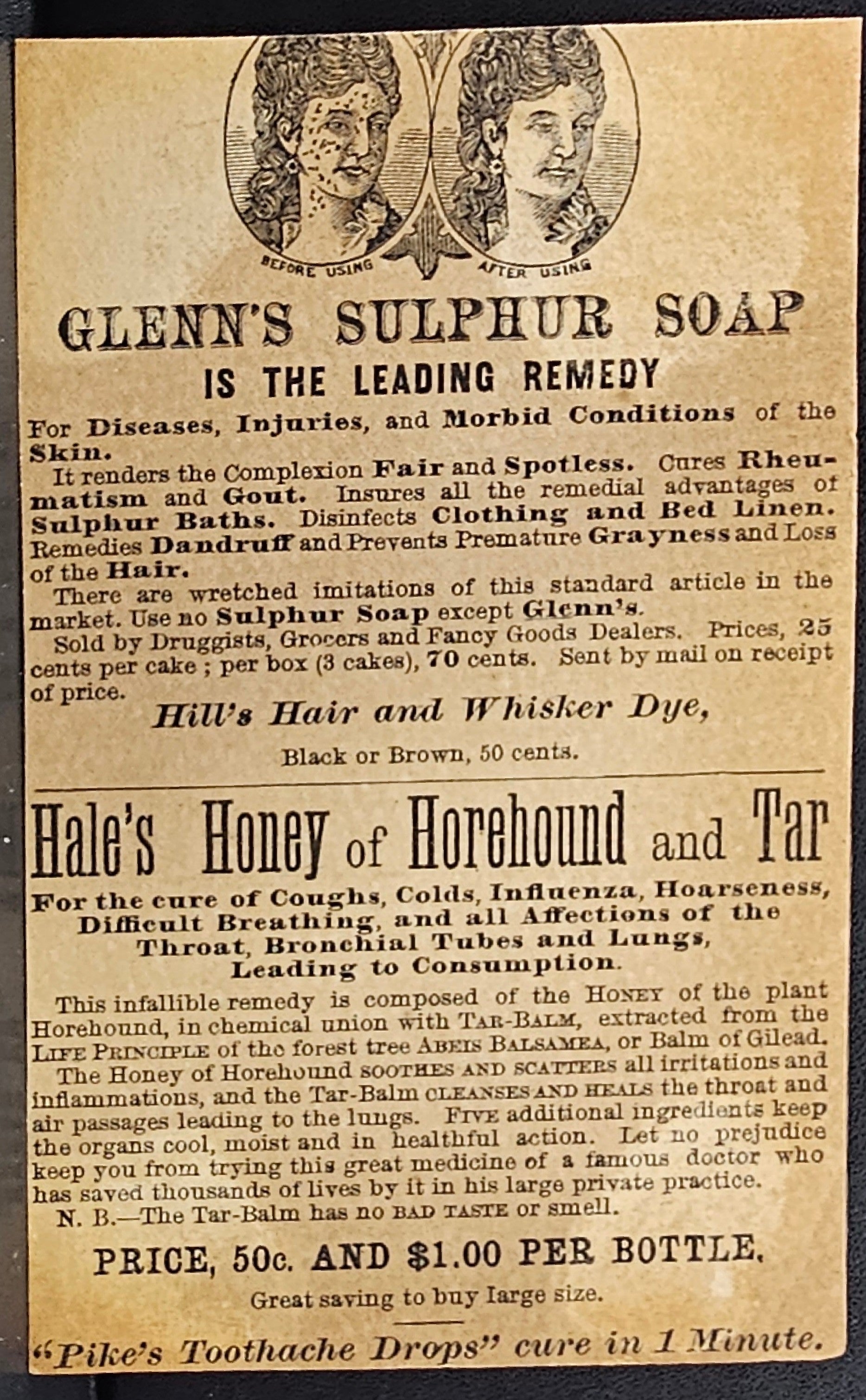The image appears to be an advertisement from around 140 years ago, characterized by its aged, brown, and stained appearance, likely from an old newspaper or a label. It features a detailed, hand-drawn depiction at the top: two images of women showcasing the before and after effects of using Glen's Sulfur Soap. The "before" image on the left shows the woman's face covered in acne, while the "after" image on the right shows her face clear of spots. The ad promotes Glen's Sulfur Soap as the leading remedy for diseases, injuries, and morbid conditions of the skin, boasting its efficacy in rendering skin transparent and healthy.

Below this, the advertisement includes a segment for Hale's Honey of Horehound and Tar, touted as a cure for coughs, colds, influenza, hoarseness, difficulty breathing, and lung infections, leading to consumption. The product details mention prices of 50 cents and $1 per bottle. The overall visual presentation is vintage, with black lettering on a light brown or beige background, framed by what looks like a dark polished wood border, typical of the era's medical advertisements often peddled by traveling medicine men.